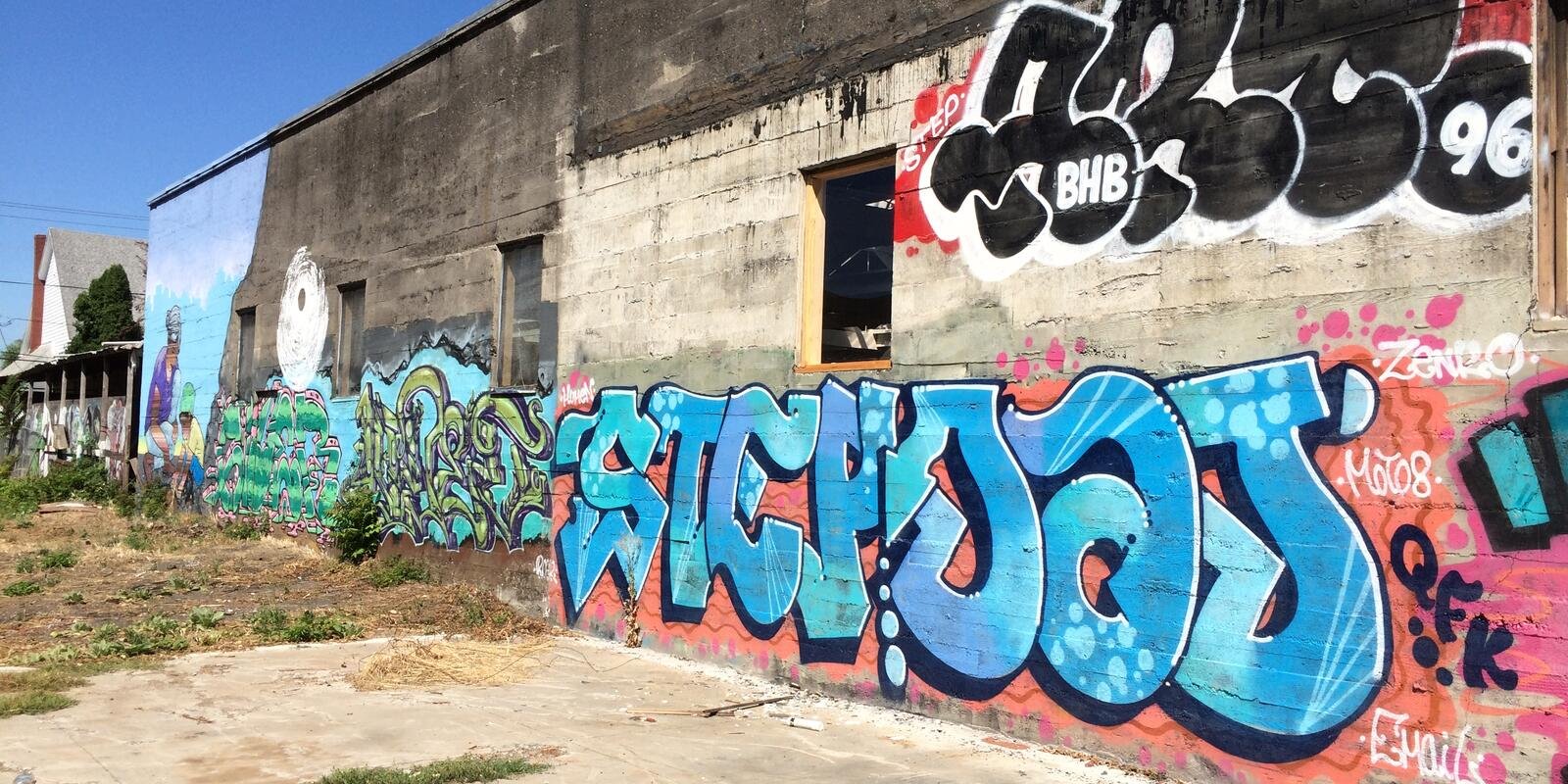The image captures a worn-down, concrete urban landscape dominated by multiple gray buildings adorned with vibrant graffiti. Centered on the facade of the largest building, the graffiti features stylized letters in blue and purple, accentuated with bubble-like designs and orange background hues. Though difficult to decipher, possible letters within the graffiti include S, T, C, and P. Above this central piece, there's a stark black spray-painted tag reading "BHB 96." Additional graffiti in black and white and smaller tags, including "Senko moto QF," surround the main piece.

On the left side of the image, green and black graffiti with a blue backdrop features a small, indistinguishable white figure, possibly a masked character. Further left, a mural depicts what looks like an African-American man bending over a woman, adding to the artistic diversity of the scene. Beyond the concrete expanse, there's an open lot with patches of grass and scattered trash, as well as visible power lines crisscrossing the sky.

In the far background, a white house with a gray roof and pillars stands amidst the urban decay, partially obscured by a tree with green foliage. The sun brightly illuminates the scene, showcasing a clear, blue sky without a cloud in sight. Concrete pavement in the foreground reveals vegetation sprouting through the cracks, indicating the area's abandoned state.